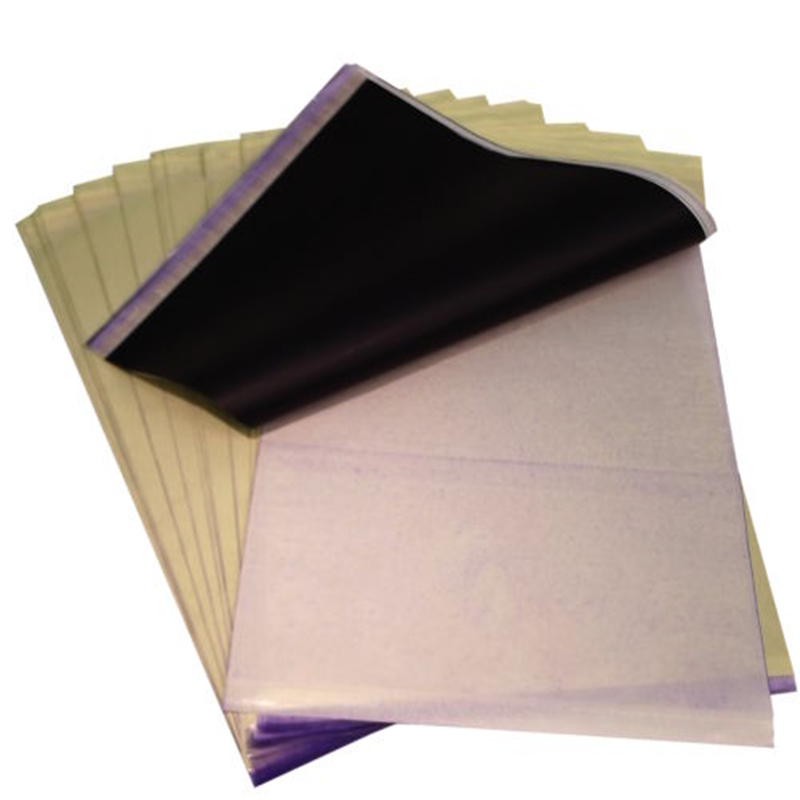This vertical image features a stack of carbon copy forms fanned out, revealing at least 10 distinct sheets. The topmost sheet is folded back, exposing the black carbon material on its reverse side, which facilitates copying written text onto the layers beneath. The forms are primarily a beige color, with the top sheet folded back to reveal a white sheet underneath. The edges of the bottom layers are tinged with a faint purple outline. This arrangement exhibits the characteristic mechanism of transfer paper, where writing on the top layer is duplicated onto the subsequent layers, thus providing instantaneous copies of handwritten documents.